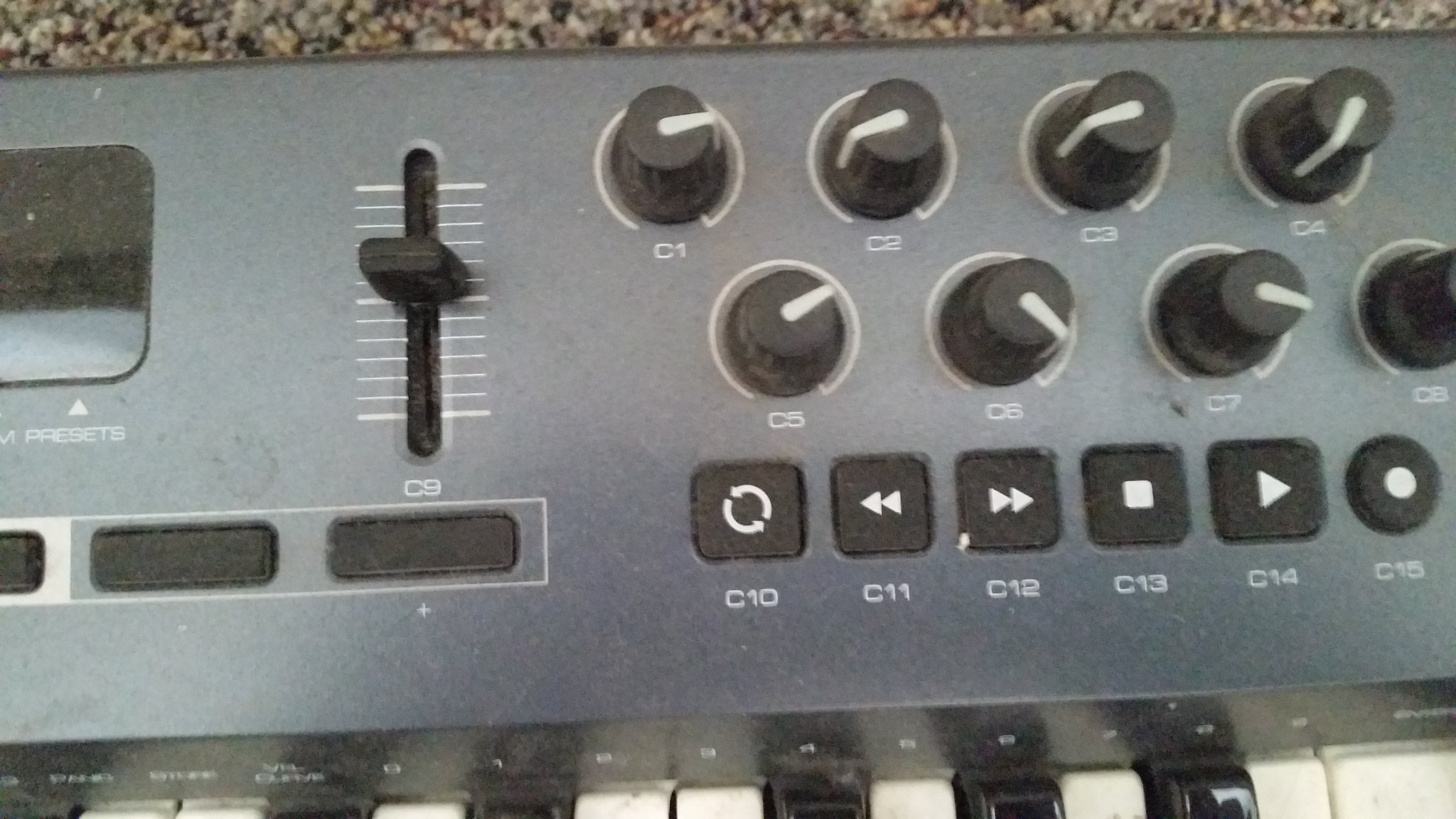This color close-up photograph captures a section of a piano keyboard with an integrated control panel, set against a background with a granular texture of brown, white, and black, possibly carpet or granite. The main focus is the control panel, which is black with a satin finish. Along the upper part of the panel are two rows of black knobs with white pointer sections, labeled C1 through C8, arranged four across the top and four across the bottom. Below the knobs is a row of five square buttons with white symbols: a circular arrow (C10), a rewind double-arrow (C11), a fast-forward double-arrow (C12), a stop square (C13), and a play arrow (C14). To the right, there is a distinct round button with a white circle, possibly for power (C15). Additionally, toward the left side of the panel, a vertical sliding dial is positioned, marked with white lines but unlabeled, along with two smaller rectangular buttons nearby. The lower part of the image reveals the top edges of the white and black piano keys, though the keys themselves are truncated by the frame. This intricate composition hints at a sophisticated musical instrument or mixer setup.